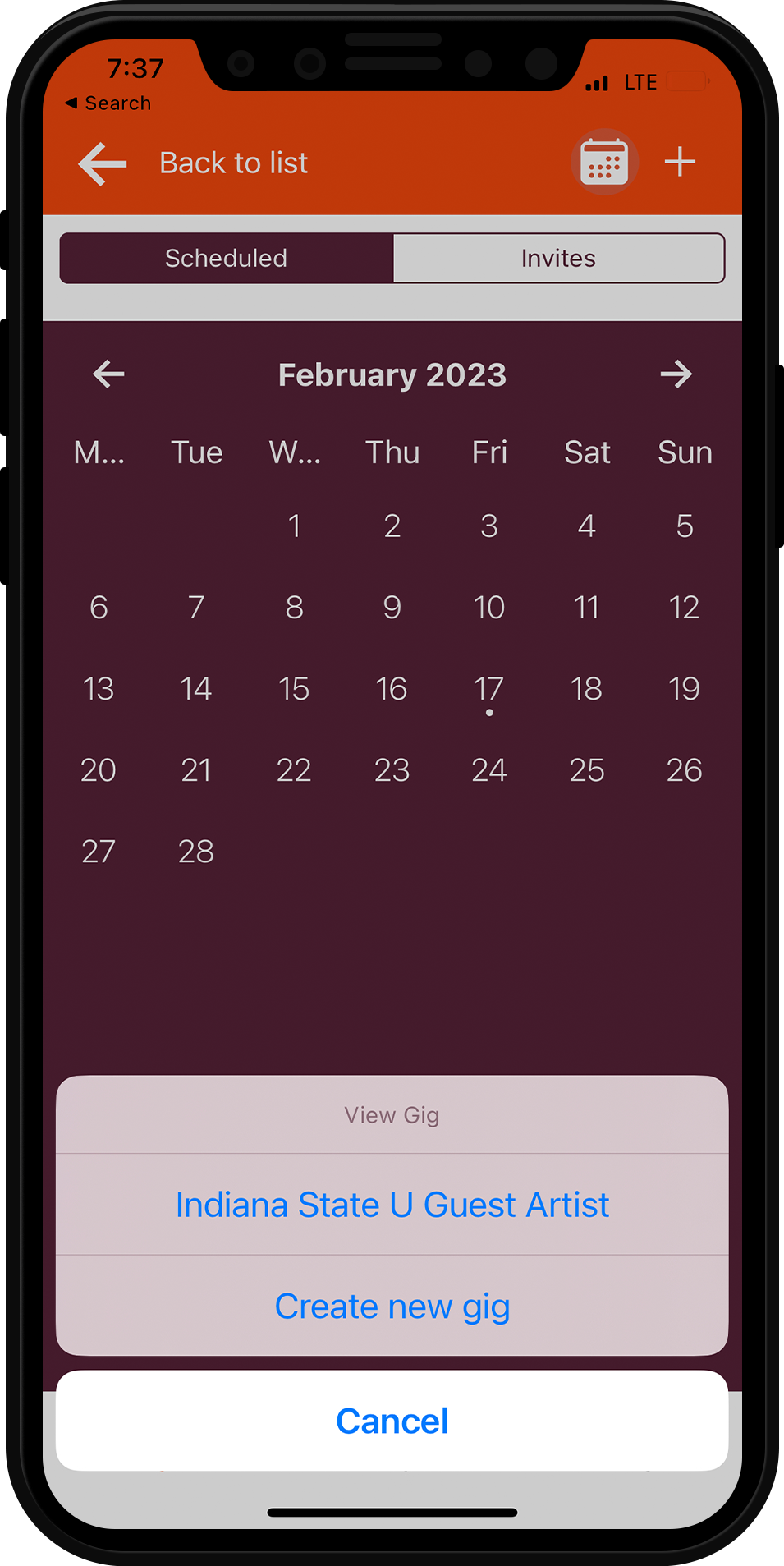The image is a portrait-oriented photograph of an iPhone encased in a black-rimmed border with rounded corners. The device features three buttons on the left side and one on the right. At the top of the screen, an orange banner displays the time "7:37" on the left, along with three bars indicating cell signal strength and the "LTE" label on the right. 

Directly below, a smaller light-orange banner includes a left-pointing arrow and the word “Search.” Beneath this, a larger white arrow also points left, accompanied by the text “Back to list.” On the right side of this banner are two icons: a calendar and a plus symbol.

The following section shows an off-white banner that contains a bisected box. The left half of the box is purple with the word "Scheduled" in white text, while the right half is the same color as the background and reads "Invite." 

The largest portion of the image features a purple background, prominently displaying a calendar for the month of February 2023.